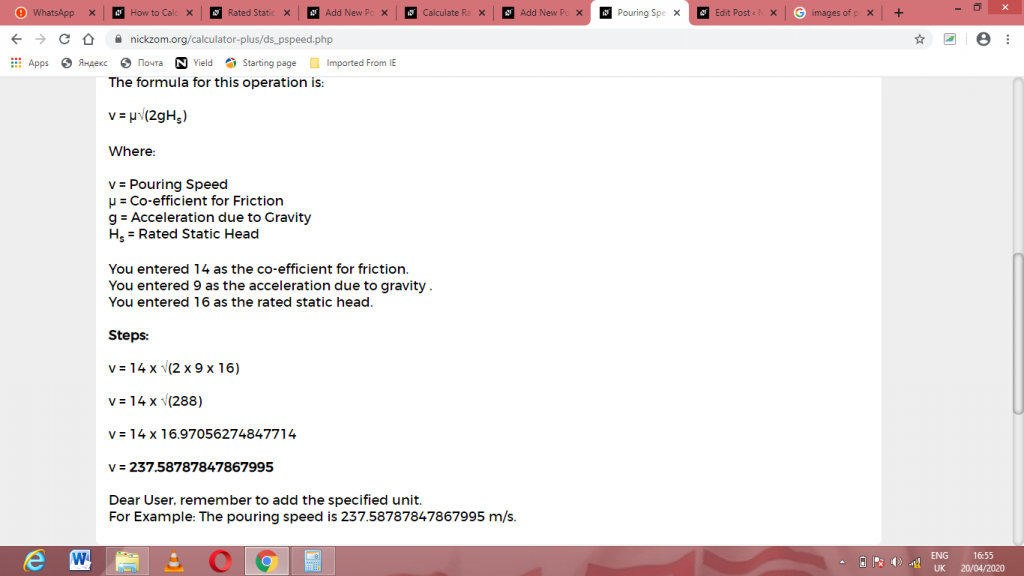The image depicts a computer screen displaying a webpage on Google Chrome. The browser has multiple tabs open, including ones for WhatsApp and another for the website nickzom.org. The main window on the screen shows a white background with black text detailing a mathematical calculation. 

The formula presented is \( v = μ \sqrt{2g h_s} \), where:
- \( v \) represents polling speed,
- \( μ \) is the coefficient of friction,
- \( g \) denotes acceleration due to gravity, and
- \( h_s \) signifies rated static head.

The user inputs provided are:
- Coefficient of friction (\( μ \)): 14
- Acceleration due to gravity (\( g \)): 9
- Rated static head (\( h_s \)): 16

The steps for the calculation are outlined as follows:
- \( v = 14 \times \sqrt{2 \times 9 \times 16} \)
- Simplifying inside the square root gives \( \sqrt{288} \)
- Thus, \( v = 14 \times 16.97056274847714 \)
- Finally, \( v = 237.58787847867995 \)

The result is \( v = 237.58787847867995 \), with an important note reminding the user to add the correct unit, such as meters per second, to the calculated polling speed.